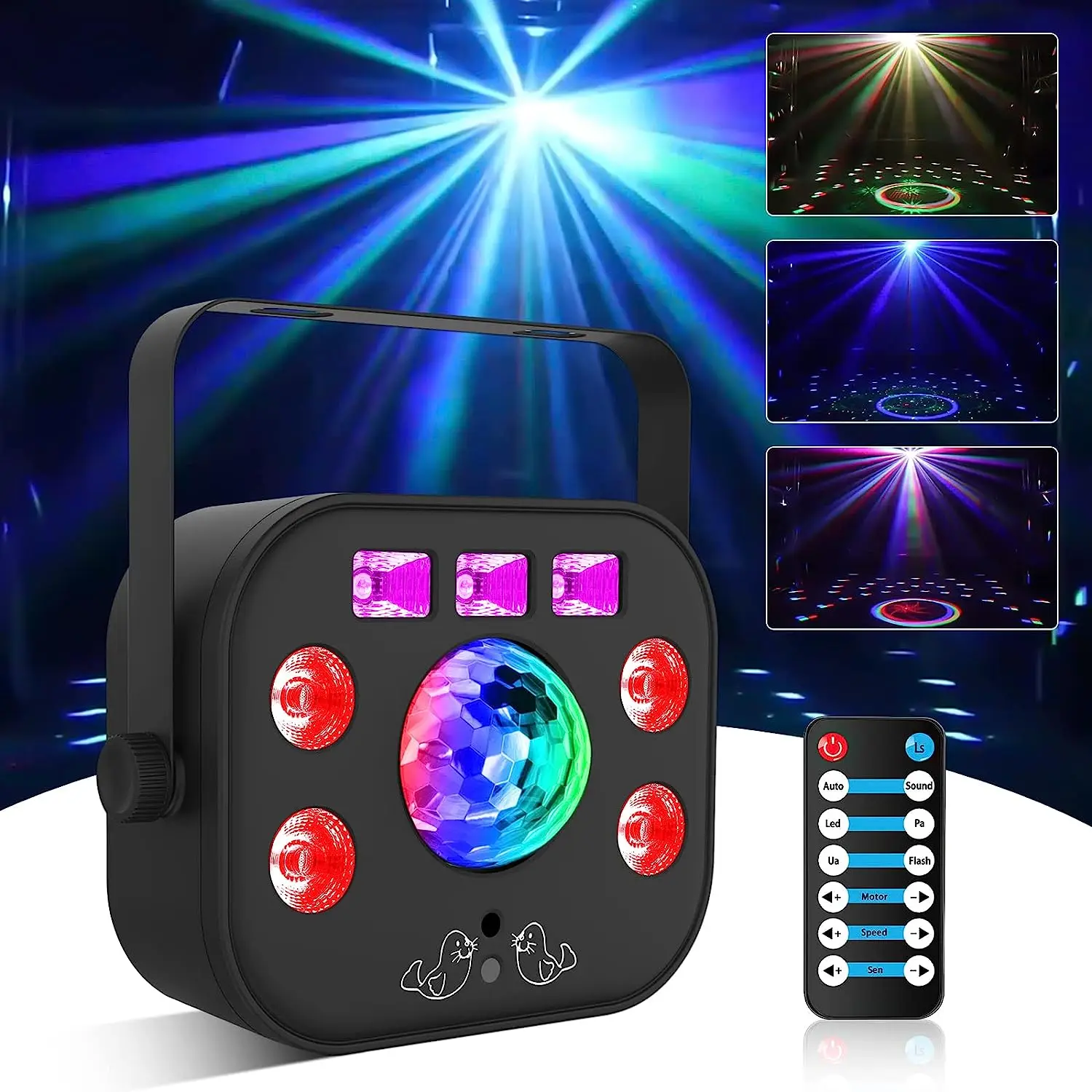This indoor photographic image features a portable disco ball and light show projector, designed for use in concerts, events, or parties. The main device is a black, square-shaped box equipped with a handle for easy transport. Its front face hosts a captivating array of lights: a central sphere emits a blend of blue and green hues, surrounded by four smaller red spheres. The top of the box is adorned with three purple rectangular elements, while the bottom exhibits two graphics depicting birds. Positioned in the lower left of the image, the projector is complemented by a remote control placed to its lower right. The remote features various functions including auto, send, LED, PA, UA, flash, motor speed, and C, along with twelve buttons arranged symmetrically. 

In the background, a spotlight emits white and purple lights, adding to the vibrant atmosphere of the scene. To the right of the main device, three smaller panels display the light effects produced by the projector: a yellow spotlight on a stage, followed by blue and purple spotlights. The composition effectively highlights the projector's versatile lighting capabilities, making it an ideal addition to any dynamic environment.